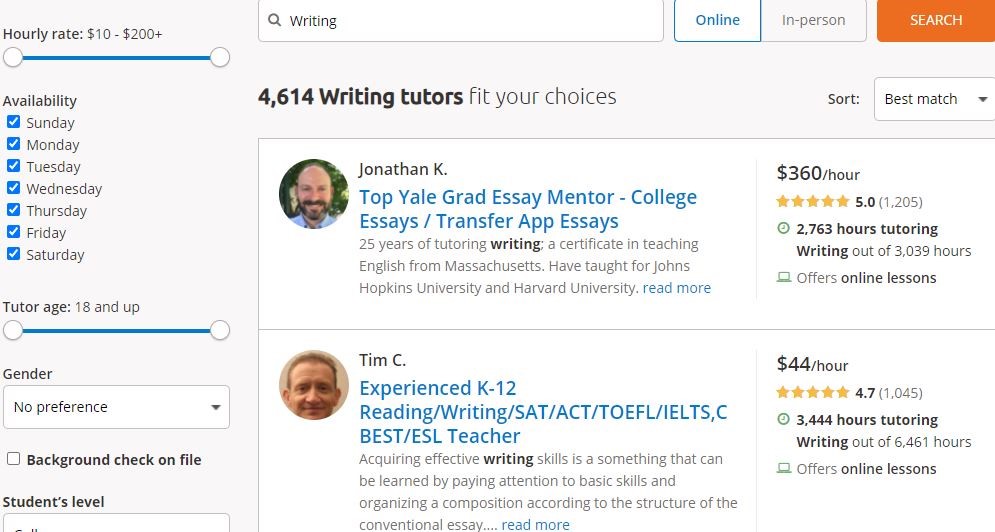The image showcases a webpage designed for finding writing tutors. At the top of the page, there is a search box with the word "Writing" pre-filled. Below the search box, there are two filter options labeled "Online" and "In-person," with "Online" being the selected option. An orange search button is also prominently displayed.

On the left sidebar, users can refine their search using various filters:

- **Hourly Rate:** Adjustable range from $10 to $200+.
- **Availability:** All days of the week are checked.
- **Tutor Age:** Set to 18 and up.
- **Gender Preference:** No preference selected in this instance.
- **Background Check:** An option to check if the tutor has a background check on file.

The main section of the page states that 4,614 writing tutors match the selected criteria. Users can sort the tutors by “Best Match.” The top result shows:

### Jonathan Kay
- **Image:** Bearded man
- **Title:** Top Yale grad essay mentor
- **Specializations:** College essays and transfer application essays
- **Experience:**
  - 25 years of tutoring
  - Certificate in Teaching English from Massachusetts
  - Teaching experience at Johns Hopkins University and Harvard University
- **Rate:** $360 an hour
- **Rating:** 5 stars based on 1,205 reviews
- **Tutoring Hours:**
  - 2,763 hours specializing in writing
  - 3,039 total tutoring hours
- **Availability:** Offers online lessons

### Tim C
- **Specializations:** Experienced with K-12 reading, writing, SAT, ACT, COEFL, IELTS, CBEST, and ESL teaching
- **Focus:** Effective writing skills through basic skills and structuring a composition according to the conversational essay
- **Rate:** $44 an hour
- **Rating:** 4.7 stars based on 1,045 reviews
- **Tutoring Hours:**
  - 3,444 hours in writing
  - 6,461 total tutoring hours
- **Availability:** Offers online lessons
- **Additional Info:** A "Read More" button for further details

This comprehensive search and filter system provides users with detailed information and multiple options to choose the most suitable writing tutor according to their needs.